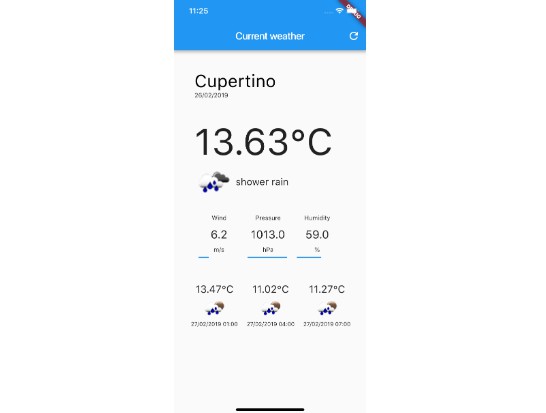A screenshot of a weather application displayed on a smartphone. The time shown is 11:25 AM. The phone has data connectivity but lacks cellular service, and the battery is fully charged. The weather app has a blue background with white font, detailing the current weather with an option to refresh the information. The top of the screen shows "Cupertino" in a white text on a blue background, with detailed information displayed on a white background with black text:

- Current temperature: 13.63°C
- Weather condition: Shower rain, depicted with an icon of a cloud with one white and one dark gray portion, accompanied by blue raindrop symbols.
- Visibility: 6.2 miles
- Atmospheric pressure: 1013.0 hPa
- Humidity: 59%

Below the main display are further weather details:

- Temperature at another time: 13.47°C on the date 2GNO2019, 
- Additional temperature readings: 11.02°C on date 27GNO2019 and 11.27°C on date 27GNO2019.

The detailed arrangement clearly outlines the current weather conditions and several specific past temperature measurements for Cupertino.